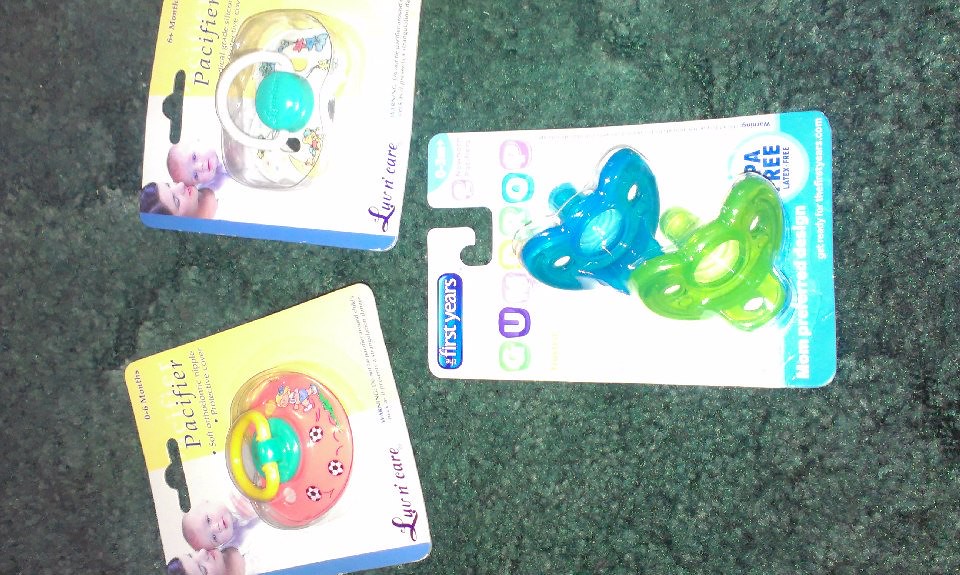The image showcases three packages of infant pacifiers arranged on a greenish-colored carpeted floor. The package on the far right is from the brand First Years and prominently features a white package with a baby blue border, labeled with "mom's preferred design," "BPA free," and "latex free." Inside this packaging are two translucent pacifiers, one blue and one green, under the product name "Gumdrop." To the left, two other pacifier packages are each adorned with the image of a woman and a baby in the upper left corner and have a yellow background stating "pacifier." The package on the far left is designed for infants aged 0-6 months and contains a pink pacifier with a girl kicking soccer balls and a yellow ring handle. The adjacent package is for ages 6+ months, featuring a white pacifier with a floral pattern and a white handle. All packages are oriented sideways with the tops to the left and the bottoms to the right, creating a cohesive display for potential sale on platforms like Craigslist, Facebook Marketplace, or eBay.